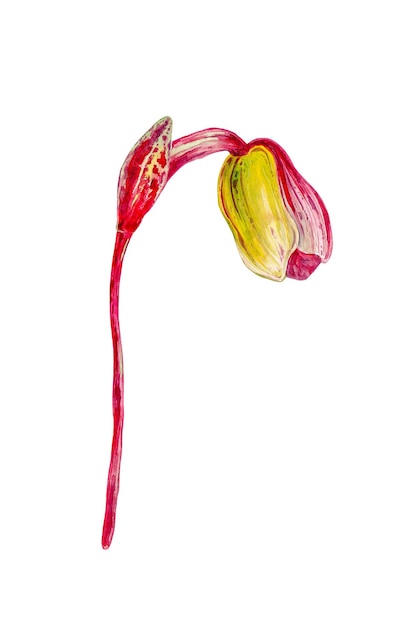The image appears to be a detailed illustration of a wilting tulip, set against a completely white background. The tulip features a red stem that curves gracefully, bending towards the bottom in the shape of a shepherd's crook. At the end of the stem, the flower head remains partially closed, its petals showcasing a mix of dark red, medium pink, and intricate white ruffled edges. One visible petal displays a combination of yellow and white hues with red veins. A single upward-pointing leaf emerges on the left side, also adorned with yellowish-white and red speckles. The overall color palette of the illustration consists primarily of reds, yellows, whites, and hints of black, emphasizing the flower's delicate, alien-like appearance.